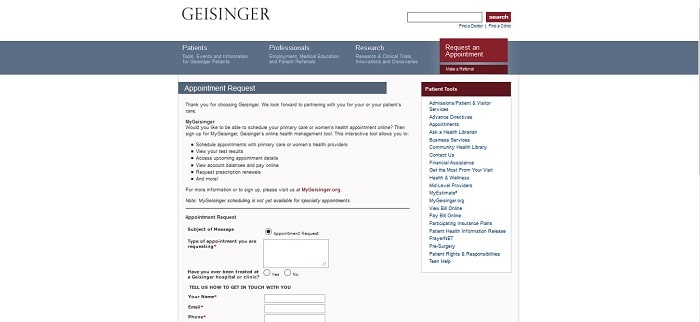The top section of the webpage prominently displays the name "Geisinger" on the left. To the right, there is a long, rectangular search bar with an accompanying burgundy-colored search button. A blue horizontal strip spans across the top of the page, featuring three clickable sections labeled "Patients," "Professionals," and "Research," each with text descriptions underneath. On the far right of this blue strip, there is a burgundy button that reads "Request an Appointment."

Below this navigational strip, the page has a clean, white background. On the left column, there is a smaller horizontal bar labeled "Appointment Request." In the right column, there is a section titled "Patient Tools," which includes a drop-down menu with various options.

The "Appointment Request" section contains a header followed by a line, a paragraph of text, a series of bullet points, more sentences, another horizontal line, and finally an input box where users can type their appointment requests.